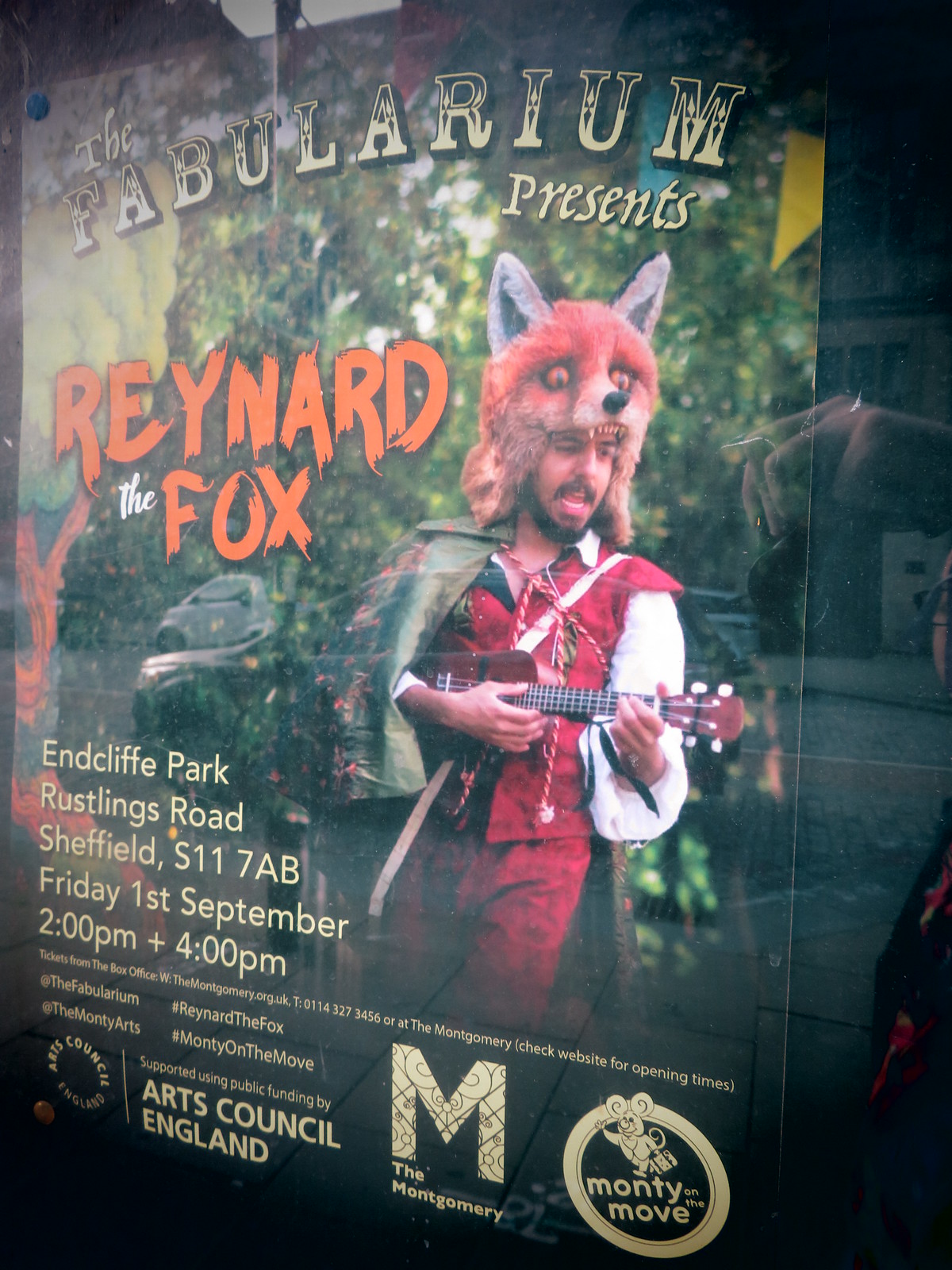The image is of a poster pinned on a surface with visible push pins on the sides. The poster advertises "The Fabularium Presents Reynard the Fox." It features a man dressed in a vintage red outfit with a green cape, donning a fox head as a hat, and playing a small stringed instrument resembling a mandolin. The background depicts a forest setting. The event details are prominently displayed: "Endcliffe Park, Rustlings Road, Sheffield, S11 7AB," scheduled for Friday, September 1st, at 2 p.m. and 4 p.m. The bottom of the poster includes several logos: "Arts Council England," "Supported using public funding by Arts Council England," "The Montgomery," and "Monty on the Move." The reflection of the person who took the photo is visible on the right-hand side.